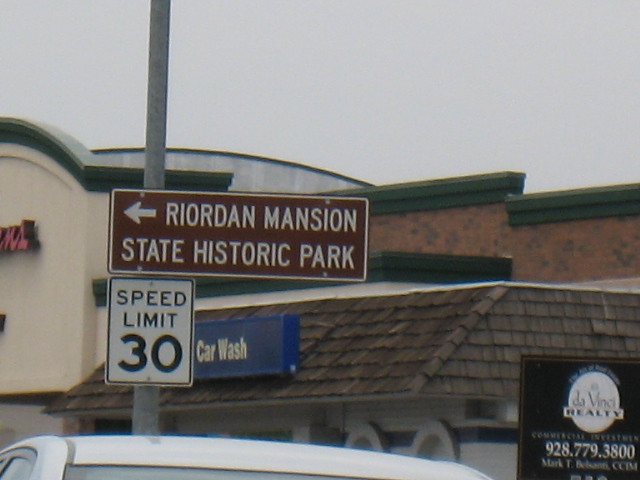In this outdoor daytime photograph taken on an overcast day, the scene is viewed above the roof of a white car positioned in the foreground. Dominating the center of the image is a plain street pole adorned with a brown rectangular sign reading "Riordan Mansion State Historic Park," complete with an arrow pointing to the left. Below this sign, a white speed limit sign indicates a limit of 30 miles per hour. In the background, to the right of the pole, an angled thatched roof features a blue sign with yellow lettering advertising a "Car Wash." On the left side of the image, the arched façade of another storefront comes into view. Further in the distance, the brick rooftop of a different building, accented with green trim, adds a layer of architectural contrast to the scene.